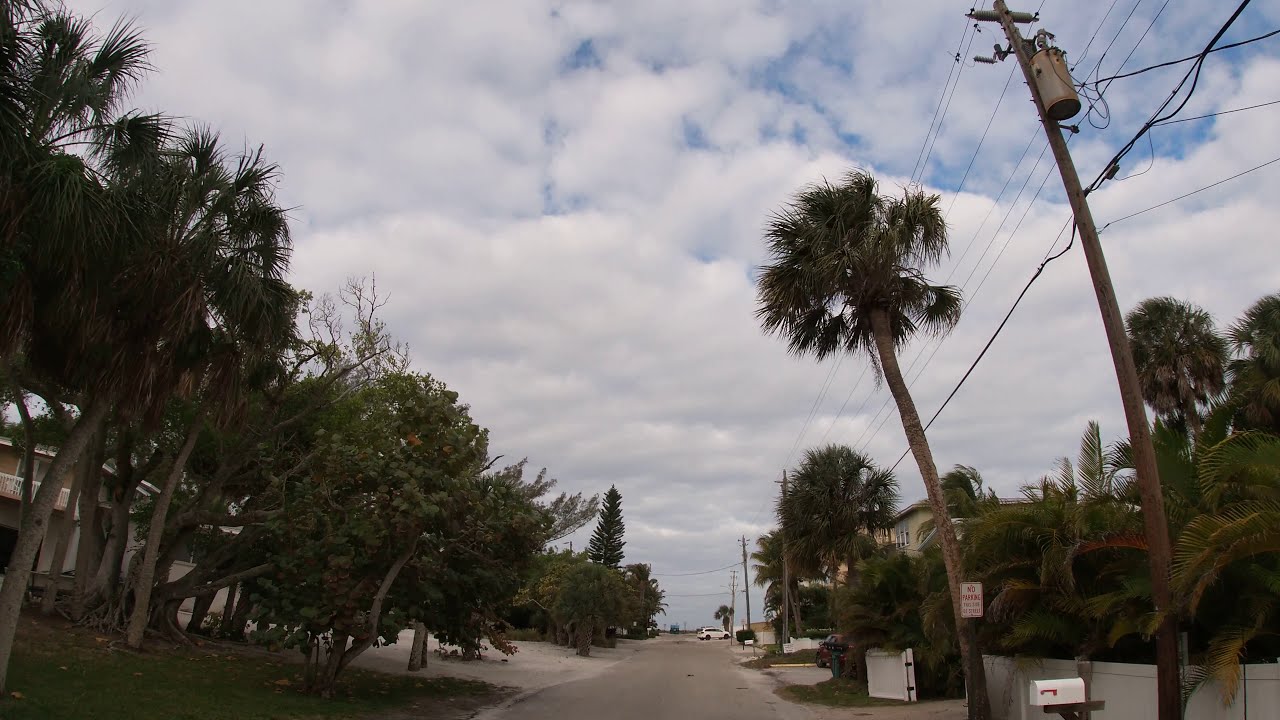The image showcases a residential neighborhood street on a cloudy day, with a mix of green, brown, tan, gray, white, red, and blue colors. The street, center at the bottom of the image, runs up the middle, flanked by various types of trees including pine trees on both sides. On the left side, there's an evergreen tree in the background, while on the right side, a prominent white mailbox with a red handle is visible near the bottom right. Both sidewalks are lined with buildings, partially obscured by the trees, and a sign on one of the trees reads "No Parking." The sky is predominantly covered with clouds, with only small patches of blue visible. There are a few vehicles parked, including a white car at the far end of the street turning right. The area also features fenced lawns and is characterized by a mix of greenery and residential structures, with telephone poles and wires running along the street.